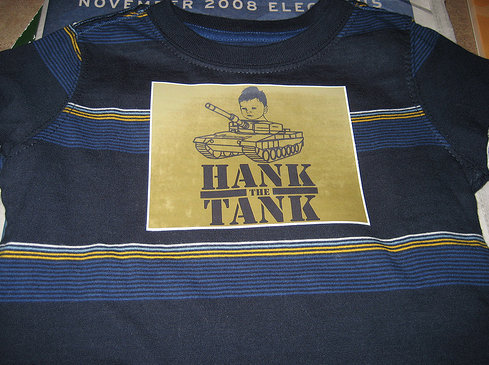The image depicts a blue t-shirt adorned with a variety of colorful horizontal stripes. The dominant color of the t-shirt is blue with alternating lighter blue, dark blue, yellow, and white stripes. Prominently featured in the center of the t-shirt is a beige or tan square that houses the phrase "Hank the Tank" in capital letters, rendered in a dark blue-gray army stencil font. Above this text, there is an illustration of an army tank with a baby's face emerging from the top, characterized by dark hair and drawn or computer-generated art. The t-shirt appears to be laid out on a surface, and in the background, partially visible, is a gray newspaper headline with the words "November 2008 elections," though not all the text is clearly readable. The surface around the shirt shows hints of brown, suggesting other items nearby.